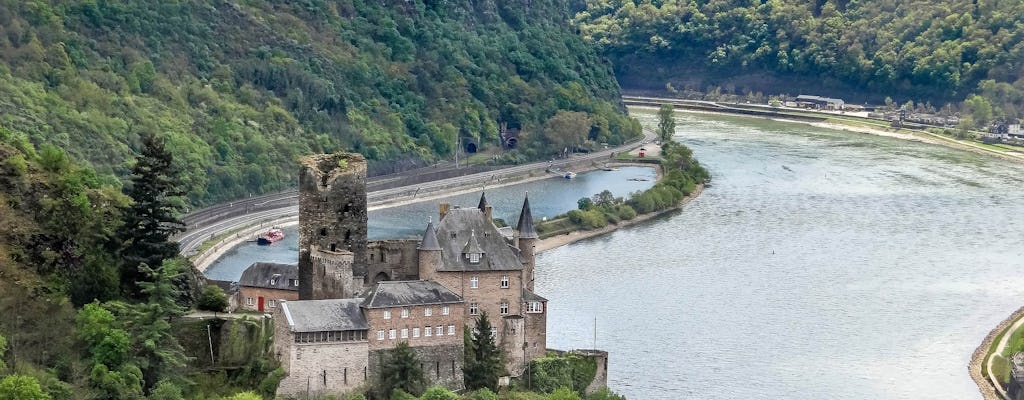This photograph presents an aerial view of a grand, stone mansion or castle set amidst a lush, green, mountainous landscape. The castle, located slightly left of center, sports several sections with varying architectural styles, including a Victorian-style structure with multiple peaks and conical roofs. Dominating the middle of the complex is an ancient cylindrical tower with a broken top, hinting at an even older ruin at the core of the estate. The left section features a large white wall, while the middle section is elevated with two rows of windows. The right section is distinguished by three tall towers and six large front-facing windows.

The castle stands on the edge of a man-made, winding canal with smooth, concrete edges, and surrounded by tree-covered cliff sides that rise majestically. The water in the canal has a dark green hue. In the background, one can see additional houses nestled beside the waterway, along with roads and potential vehicles. These elements deepen the sense of the estate’s integration into the surrounding verdant, mountainous terrain. The scenic beauty is accentuated by abundant evergreen trees and green bushes that blanket the hillsides around the castle, adding to the picturesque quality of the image.